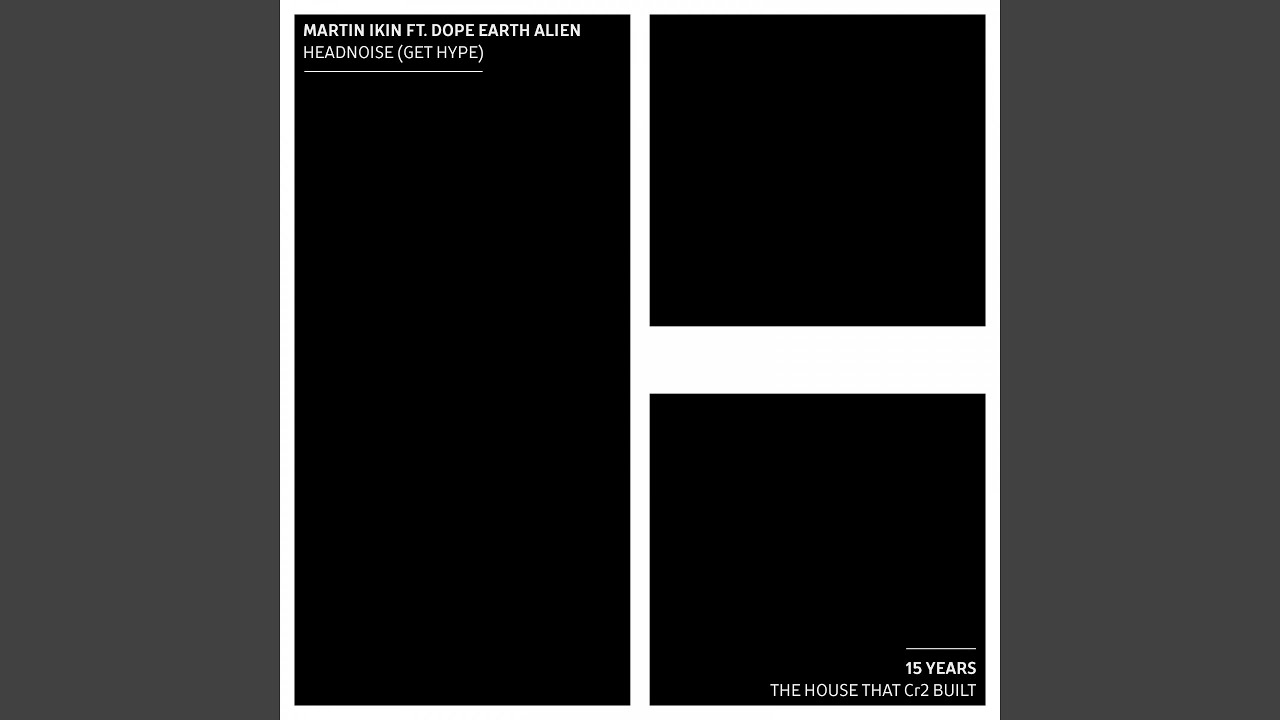The image displays a screen featuring a series of five vertical boxes and rectangles in varying shades of black and gray. The boxes exhibit different heights but are uniformly center-aligned on the page. The extreme left and right boxes are identical, extremely dark gray, and very narrow, stretching the entire height of the screen. These two boxes create a symmetrical frame on either side.

Adjacent to the box on the far left is a second box that mirrors its shape but is slightly shorter and completely black. Positioned at the top left of this box is a cluster of letters, bolded and capitalized, with a thin gray line underneath.

Further right, there are two additional rectangular boxes of identical length to the second left box, separated by a narrow gap. These shapes contribute to the overall balance and symmetry of the design. The subtle variations in color and alignment create a precise and structured composition.